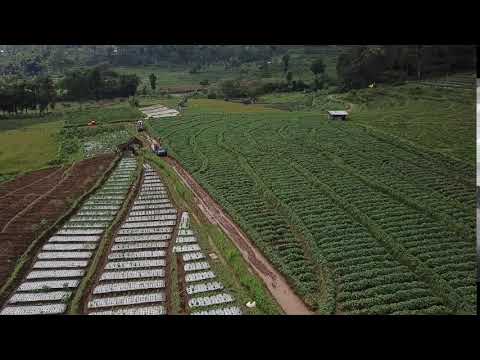This image captures a rural farmland scene taken from a high vantage point, most likely atop a hill, during the daytime. The photograph appears slightly blurry and of low resolution, lending it a somewhat indistinct quality. Central to the image, a brown, possibly muddy dirt road runs vertically, dividing the scene into two distinct halves. Along this road, a couple of vehicles are visible, suggesting some activity.

On the left side of the road, the field is characterized by dark brown, bare dirt, indicating a freshly plowed area either prepped for planting or newly planted. This side also features regions with white coverings, likely protective tarps over seedlings or pots.

In contrast, the right side of the image boasts rows of vibrant green crops, although the specific type of vegetation remains unidentified. Further up, in the upper portion of the scene, the landscape includes additional fields, small buildings, possibly a white house or shed, and an assortment of tall trees. The overall terrain is slightly hilly, contributing to the layered appearance of the fields, which resemble parallel railroad tracks from this angle.